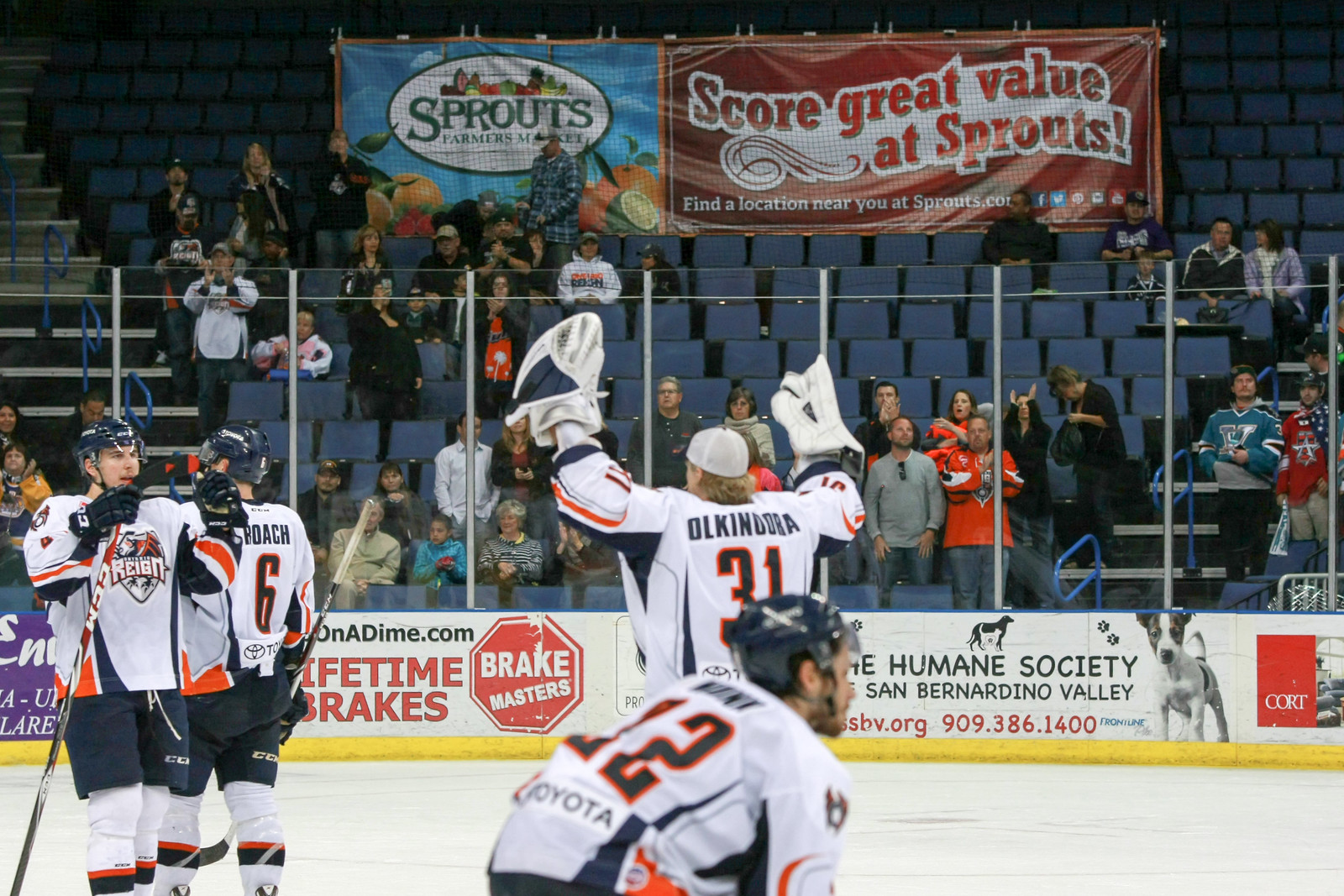In a vibrant hockey arena, four players clad in blue and orange uniforms with white pants, highlighted by red and black at the bottom, are seen on the ice, seemingly celebrating or possibly warming up for their next move. One of the players, notably the goalie, stands out with his white helmet and raised pads. Adorning their jerseys is the name "REIGN," indicating their team affiliation. Above them, the arena is lined with various advertisements. Dominantly, two Sprouts Farmers Market banners catch the eye—one blue featuring images of assorted vegetables, and the other red with the slogan, "Score great value at Sprouts. Find a location near you at Sprouts.com." Additionally, there are ads for "On a Dime," "Lifetime Breaks," "Breakmasters," and a notable sign for "The Humane Society of San Bernardino Valley," complete with a dog image, website “ssmed.org,” and phone number “909-386-1400.” The stadium seats behind the action have sparse attendance, with a few scattered spectators intently watching the scene on the ice.